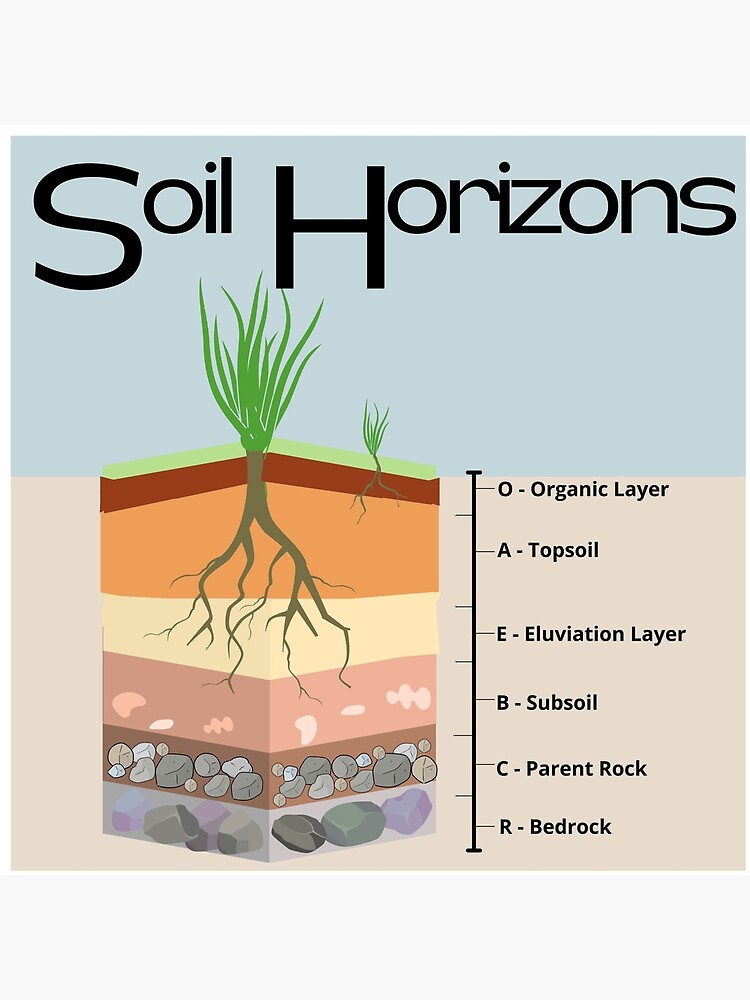The image is a detailed diagram showcasing the cross-section of soil layers, titled “Soil Horizons” in black font at the top. A green-leaved plant sits atop the soil with its brown roots delving deep. To the right, labels define each soil layer: O (Organic Layer), A (Topsoil), E (Eluviation Layer), B (Subsoil), C (Parent Rock), and R (Bedrock). The layers exhibit distinct colors—green and red for the Organic Layer, orange for the Topsoil, beige or cream for the Eluviation Layer, pink for the Subsoil, gray pebbles for the Parent Rock, and larger gray pebbles for the Bedrock—visually emphasizing the vertical arrangement of soil horizons. This graphic serves as an educational tool to illustrate the stratification and composition of different soil types.